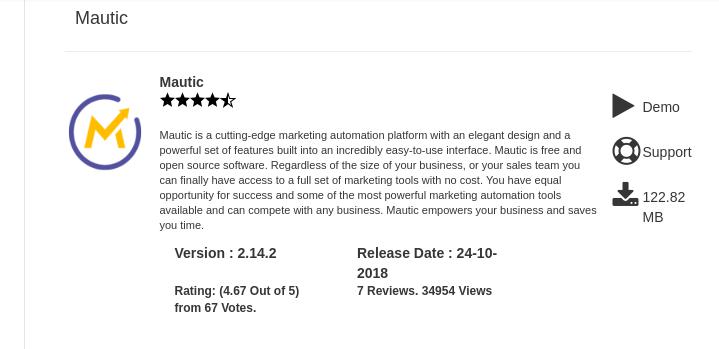Here is the cleaned-up and detailed caption:

---

**Mautic: Premium Software Rating Snapshot**

This screen capture showcases a rating for Mautic, a marketing automation platform, with an impressive score of 4.67 out of 5 stars based on 67 votes. The rating illustration features an 'M' icon accentuated by an upward-trending arrow, symbolizing growth and success.

**About Mautic:**

Mautic stands out as a cutting-edge marketing automation platform, renowned for its elegant design and powerful suite of features. The software is celebrated for its incredibly user-friendly interface, making it accessible to businesses of all sizes. As a free and open-source tool, Mautic provides equal opportunities for success by ensuring that every organization, regardless of its size or sales team strength, can access a comprehensive set of marketing tools at no cost.

Mautic is not just about affordability; its robust automation capabilities empower businesses, allowing them to save valuable time and compete effectively in the market. This marketing automation platform exemplifies the combination of elegance, power, and accessibility, setting a high standard in the industry.

---